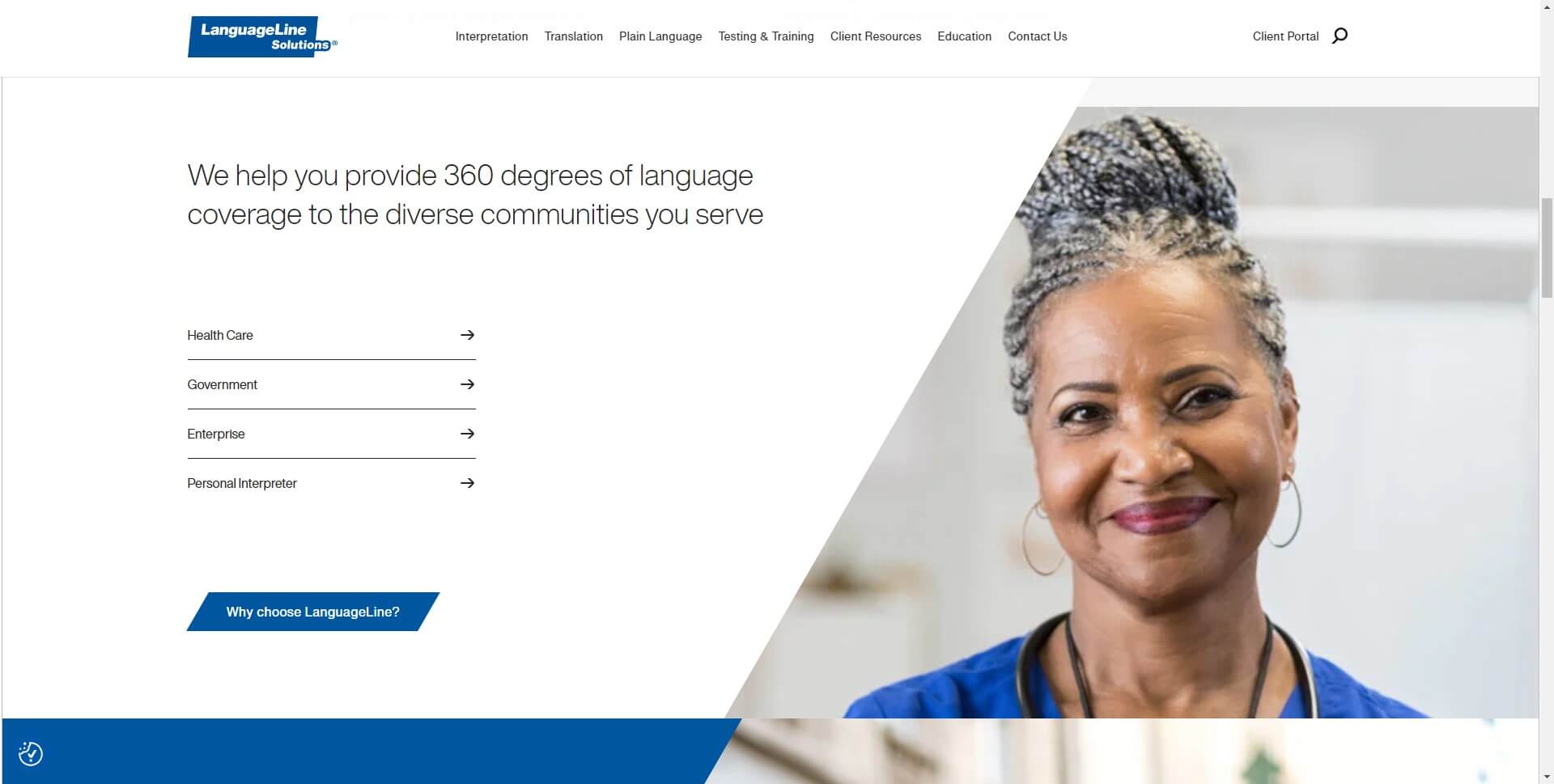In the screenshot, a woman with black and gray braids is depicted. She appears to be wearing scrubs, suggesting she might be a nurse. The image prominently features a magnifying glass and what seems to be a clear portal. The text on the image indicates the message "We help you provide 360 degrees of language coverage to the diverse communities you serve." Additionally, the term "health care" is visible, although the "C" may be cut off, along with the phrase "personal interpreter." A blue rectangle with white text reads "Why choose Language Line." To the right of the image, a gray scroll bar is seen, indicating that more information might be available beyond the visible area.